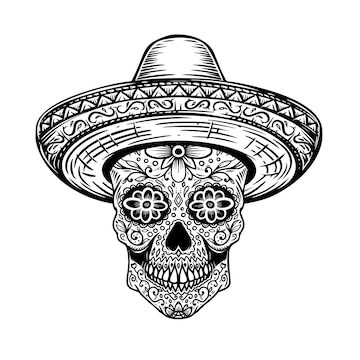This detailed line art portrays a skull adorned with an intricate sombrero, rendered entirely in black ink against a white background. The artwork reflects a Mexican cultural style, akin to Cinco de Mayo or Día de los Muertos (Day of the Dead). The skull showcases elaborate decorative elements, including flower-shaped eyes and a prominent flower located on the forehead beneath the brim of the sombrero. Additional detailing includes leaves, symmetrical curly lines, and swirling stems that extend from the cheekbones, creating a tapestry of ornate patterns. The nasal cavity is represented by an upside-down heart shape, and the jawline features symmetrical teeth. The sombrero is embellished with designs resembling S's, backwards S's, and triangles, adding to the overall intricate aesthetic of this monochromatic line drawing.